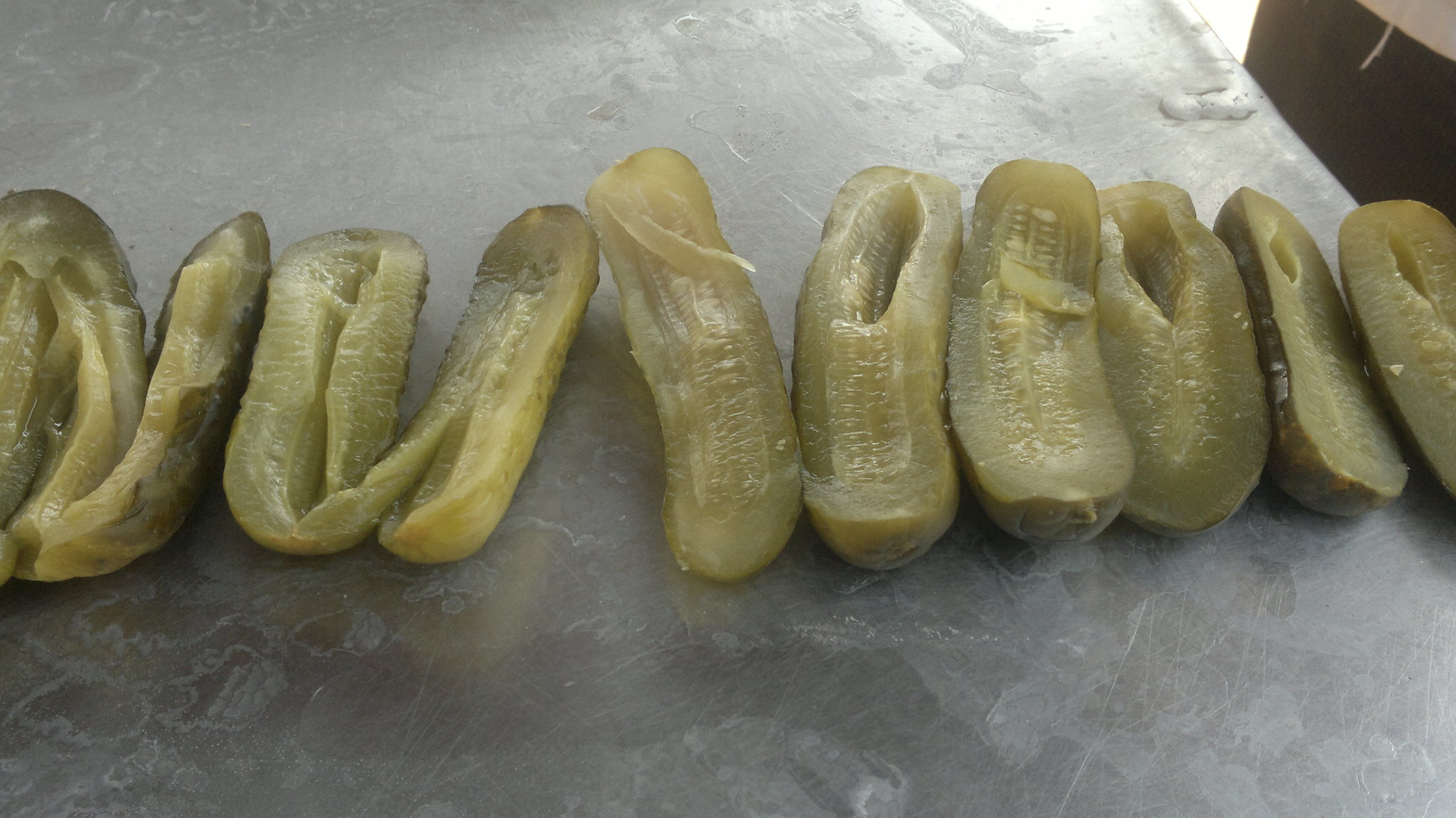This image captures six large, mature pickles sliced in half and arranged on a white, marbled countertop. The pickles rest with their insides facing up, revealing light green flesh dotted with small seeds. While some halves are split further into quarters, the others remain more intact. The pickles exhibit a bumpy, dark green exterior contrasted with smooth, moist interiors. You can also observe small puddles of water on the countertop, contributing to the fresh and glistening appearance of the pickles. The upper-right corner of the image features the edge of a brown table, adding a contrasting element to the scene. The overall atmosphere suggests freshly prepared pickles laid out in a meticulous and slightly rustic fashion.